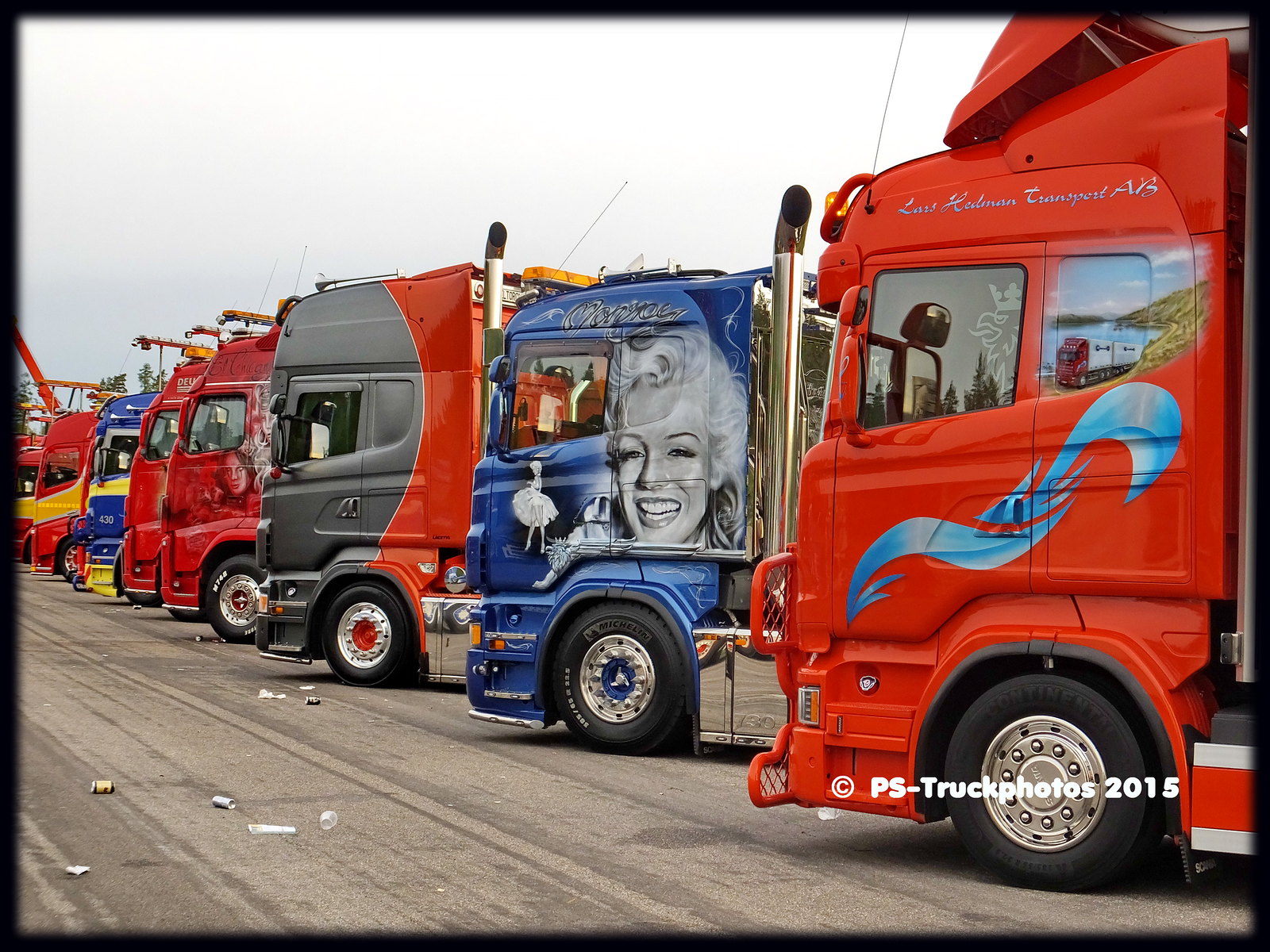This photograph depicts a row of eight large trucks parked at an angle in a gray, litter-strewn parking lot. The sky above is overcast, casting a muted light over the scene. Starting from the left, the first truck is striking with its red cab adorned with a blue swirly design stretching over the cab to the back window, which features an image of a truck on a winding road. The driver's window is decorated with a picture of a rooster, and the cab is labeled "Lois Hedman Transport AB."

The next truck, slightly shorter in height, has a blue cab with silver detailing and a detailed image of Nancy Sinatra in a ballerina skirt painted on the door. This truck also prominently displays the name "Nancy." 

Following is a gray and red truck with a semicircular grayish pattern extending over the cab. 

The fourth truck is dark blue, showcasing a black-and-white portrait of Marilyn Monroe, including her iconic white dress. 

Subsequent trucks further down the line include another red truck, a blue and yellow one, and another red truck with a face that is hard to distinguish due to the distance. The final trucks are difficult to make out clearly. 

The scene also includes scattered litter and empty drink cans on the tarmac, with a watermark in the bottom left corner that reads "PS Truck Photos 2015," capturing a moment in time within this industrial setting.